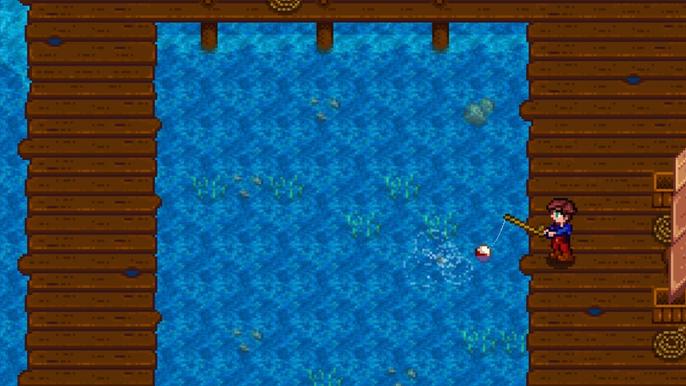The image appears to be a nostalgic depiction from an old-school, 8-bit video game set on a fishing pier. The scene is viewed from above, showcasing a wooden dock constructed from brown planks that form a rectangular pool in the center, filled with blue water. The dock is supported by visible pillars and is bordered by various walkways. The water below is dotted with green seaweed-like formations and vague images of fish, possibly in schools of three. To the far right stands a pixelated character, likely a young boy with brown hair and blue eyes, dressed in a blue shirt, red pants, and brown shoes. He is actively fishing with a stick fishing pole, which has a distinctive red and white bobber at the end of the line. Adjacent to him are some pixelated elements that might represent storage bins, rope, or an awning, adding to the fishing pier ambiance.